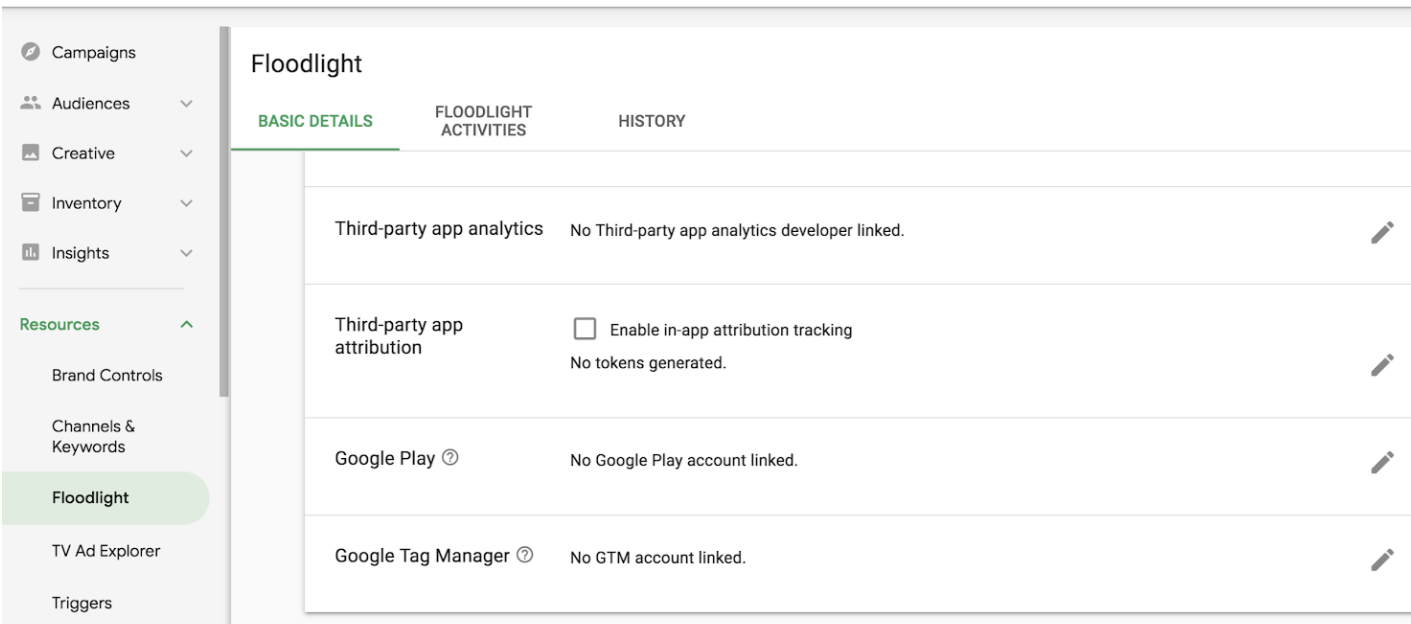This is a detailed screenshot from an unidentified website interface, showcasing a digital analytics or advertising management tool. The screenshot captures a vertical navigation menu on the far left with multiple listed sections: Campaigns, Audiences, Creative, Inventory, Insights, Resources, Brand Controls, Channels and Keywords, Floodlight (which is currently selected), TV Ad Explorer, and Trigger.

To the immediate right of the menu, the top of the interface features the heading "Floodlight," under which are tabs labeled Basic Details, Floodlight Activities, and History. The tab Basic Details is selected.

Under the Basic Details section, several features and settings related to third-party app analytics and attribution are displayed:

- "Third-party app analytics: No third-party app analytics developer linked."
- "Third-party app attribution," accompanied by an unchecked box labeled "Enable in-app attribution tracking."
- "No tokens generated."
- "Google Play: No Google Play account linked."
- "Google Tag Manager: No GTM account linked."

Each option listed under these settings has an icon of a pencil situated diagonally, slanting downwards to the left, implying that the settings are editable.

The overall image is a clear, wide interface devoid of any photographic elements. It includes no images of people, plants, flowers, trees, automobiles, or airplanes. The focus is entirely on the structured layout and textual information presented within the web interface.